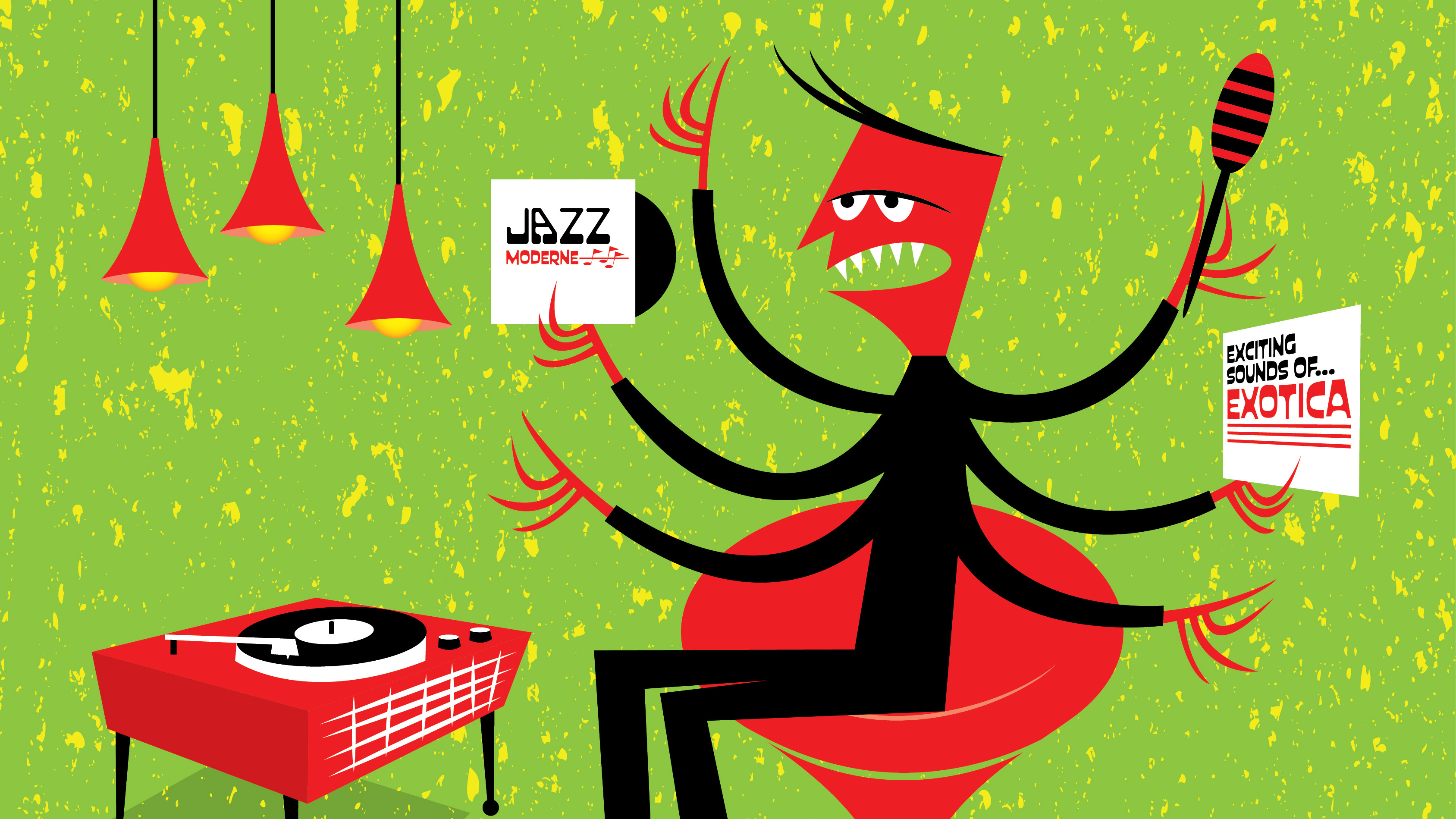The artwork depicts a cartoonish, edgy scene with a lime green background speckled with white. At the center of the image, slightly to the right, is a red-skinned creature with a flat-topped head and sparse black hair. Dressed entirely in black, the creature has six spindly arms, each with four elongated fingers. The creature's sharp, white teeth are bared in an unsettling grin. It is seated in a red, bowl-shaped chair.

The creature's arms are busy with various objects: the top left-hand holds a record sleeve labeled "Jazz Modern" with a black and white cover, a vinyl record peeking out. The middle right hand grasps another record sleeve, this one emblazoned with "Exciting Sounds of Exotica" in underlined red font. The top right hand shakes a maraca, while the other hands remain free.

In the left foreground of the image stands a red record player with black legs. It plays a record, the tonearm and needle strikingly white against the darker components. Above the record player, three red, triangular sconces with glowing yellow bulbs hang at varying heights from black cords, illuminating the surreal scene below with a warm light. The creature's dark pinkish face, the red furnishings, and the contrasting green background contribute to a whimsical yet eerie atmosphere.